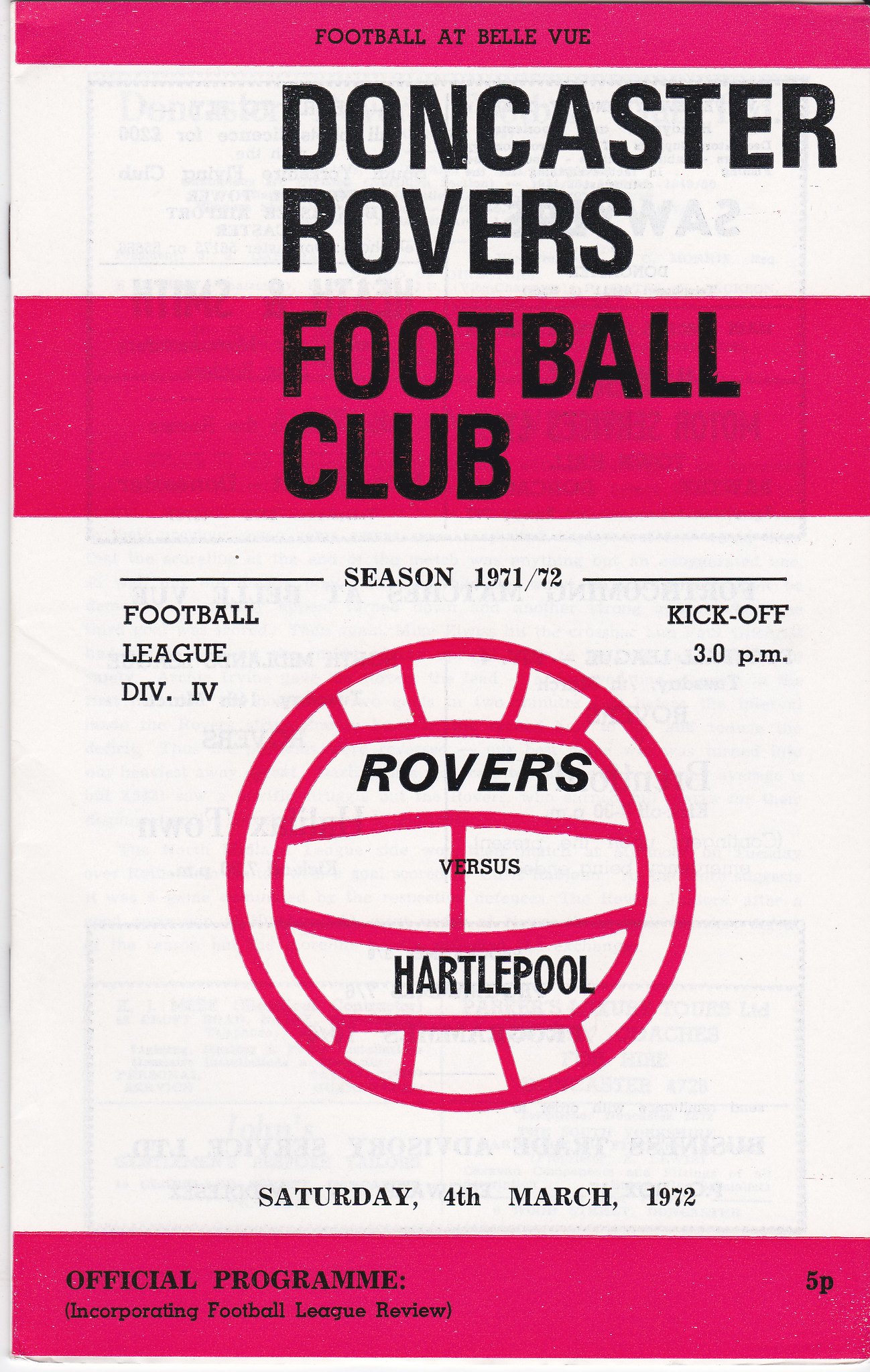The cover of the sporting program, primarily adorned in a pink and white color scheme, features distinct pink and white stripes. At the top, encased in a pink stripe, the text "Football at Bellevue" is inscribed in small black ink. Below that, nestled within a white stripe, "Doncaster Rovers" is prominently displayed in large black letters. Continuing downward, another pink stripe showcases "Football Club" also in large black letters. The central focus of the design is a pink and white soccer ball illustration, within which "Rovers versus Hartlepool" is prominently highlighted. Above the ball, the text "Season 1971-72" is neatly positioned, flanked by black lines. On the left side in black text, the words "Football League Division IV" appear, and on the right, "Kickoff 3.00 PM" is noted. Beneath the soccer ball illustration, the date "Saturday, 4th March, 1972" is clearly indicated. At the very bottom, another pink stripe holds the phrase "Official Program Incorporating Football League Review," with an added detail on the right side showing "5p."